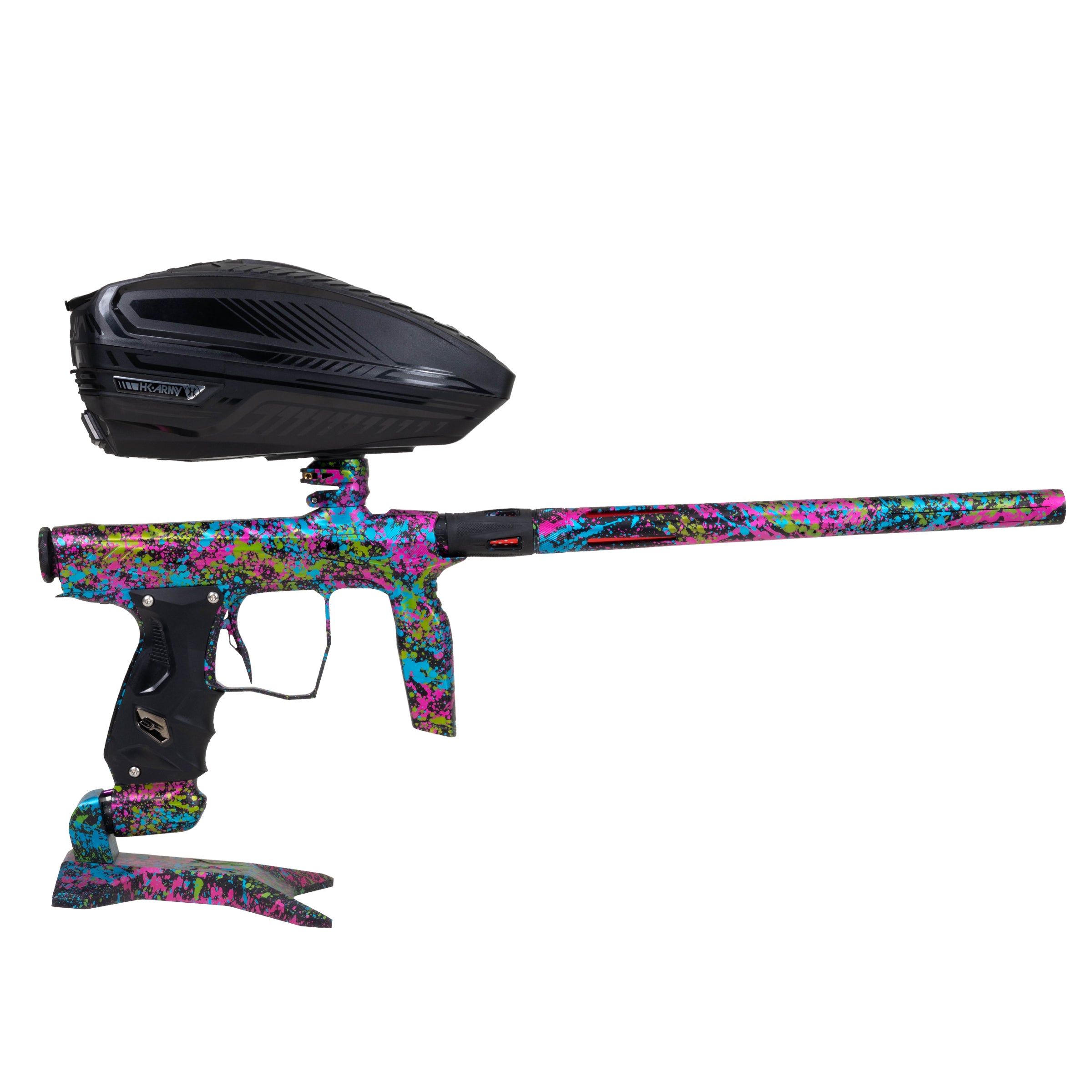The image features a multicolored paintball gun with a striking array of colors, including neon pink, neon green, neon blue, gray, white, red, black, purple, and yellow. The gun is positioned from left to right, with the barrel extending outward. At the top, there's a large, helmet-like black container, presumed to store either paintballs or gas for propulsion. The handle is black, designed to be gripped with one hand, while another section forward of the trigger provides an additional grip. The gun also incorporates a foot-like stand feature, allowing it to be set on the ground or a bench for stability. The overall style of the gun is psychedelic, with its vibrant, spray-paint-like mix of colors creating a visually captivating effect.